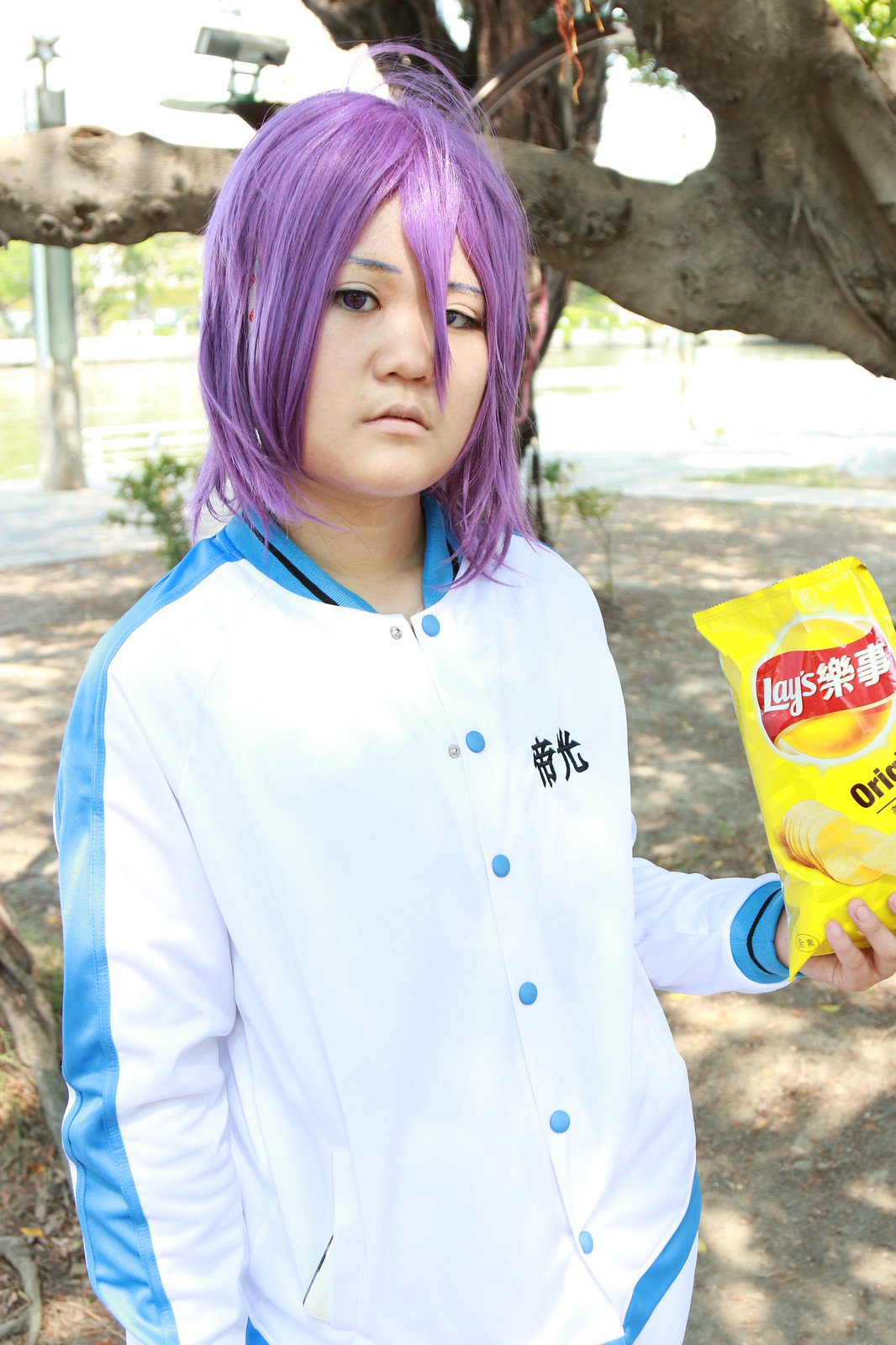This outdoor photograph is centered on a young woman with shoulder-length lavender hair, styled in a short, fashion-forward cut. She is wearing a distinctive long-sleeve, majority white varsity jacket featuring light blue buttons and aqua trim, which includes a stripe running down the outside of each arm. The jacket also bears black Asian characters on the upper left side, adding an element of detail and intrigue to her attire.

The woman stands under the dappled shade of a large tree, the branches of which frame the top of the image and cast interesting shadows and light patterns below. In her left hand, she holds a small, yellow bag of Lay's potato chips, which prominently displays a potato chip graphic and is marked with Japanese writing, adding another layer of cultural detail.

She gazes directly at the camera with a mild frown, creating a candid and captivating expression. Behind her, the scene extends into a background of shaded earth and distant trees, with a street faintly visible further back, enhancing the natural, serene outdoor setting.